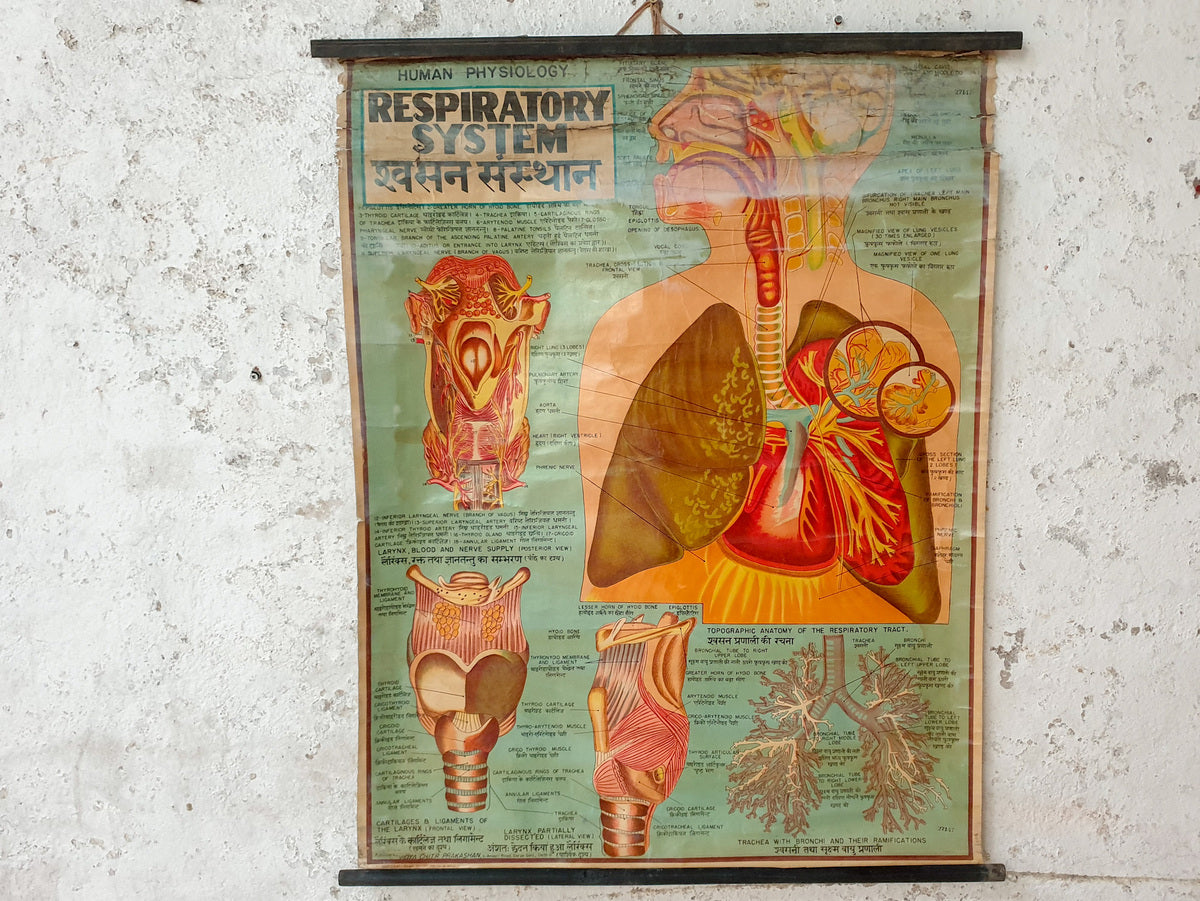The image captures an old, worn-out informational poster, likely from a doctor's office, titled "Human Physiology: Respiratory System." The poster is mounted on a wall with a marble-patterned background, characterized by white and grey flecks. The title is prominently written in black font, and beneath it, there appears to be some additional text in a hieroglyphic or South Asian language. The central illustration features a detailed diagram of the upper half of a human body, focusing on the respiratory system. It shows a male figure with his head turned to the left, revealing internal organs including the lungs, heart, trachea, and pharynx. The trachea and spinal cord are clearly visible, as well as various arteries, veins, and respiratory tubes extending into the head and brain. Surrounding the main figure, there are several close-up illustrations of individual organs and parts of the lung, labeled with detailed text that is mostly illegible due to its small size. The color scheme of the diagram background is a subtle turquoise, contributing to the vintage feel of the poster.